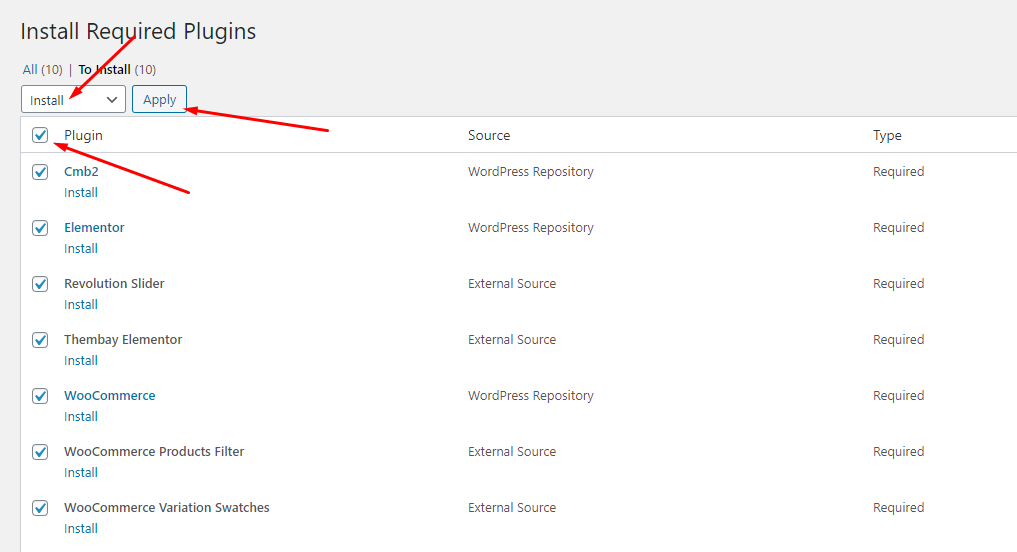The background of the image is light gray. At the top left corner, there is black text that reads "Install Required Plugins." Directly below, in blue text and enclosed in brackets, is the number "10," alongside black text stating "to install" also enclosed in brackets, indicating there are 10 plugins to install. A red arrow extends from the "required" text to a drop-down menu currently displaying "install." Another red arrow on the right points to an "apply" button that has blue text, a blue outline, and a light blue fill.

There is also a red arrow pointing at the first tick box in the "Plugin" column. The "Plugin" column is the first category, followed by "Source" in the middle, and "Type." Every entry in the "Type" column is labeled as "Required." The "Source" column lists the origin of each plugin, starting with:

1. WordPress Repository
2. WordPress Repository
3. External Source
4. External Source
5. WordPress Repository
6. External Source
7. External Source

The "Plugin" column lists the following plugins alongside the word "install":

1. CMB2
2. Elementor
3. Revolution Slider
4. Thimble Elementor
5. WooCommerce
6. WooCommerce Product Filter
7. WooCommerce Variation Swatches